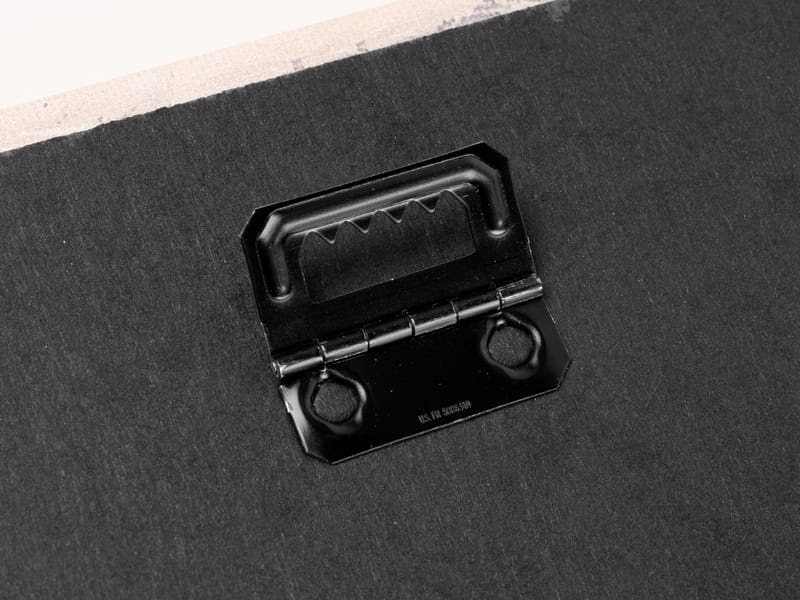This photograph features a metallic object resembling a component of a cabinet hinge. The black-painted base of the object includes two screw holes, designed to anchor it securely. Extending upward from the base is a hollow, rectangular structure crowned with four small teeth-like projections. The object rests on a black material, possibly a piece of fabric or rubber. Beneath this material is a white surface, possibly paper, with some faded or smudged text visible. The intricacies of the hinge and the contrasting background elements create a visually intriguing composition, highlighting the mechanical details of the object.